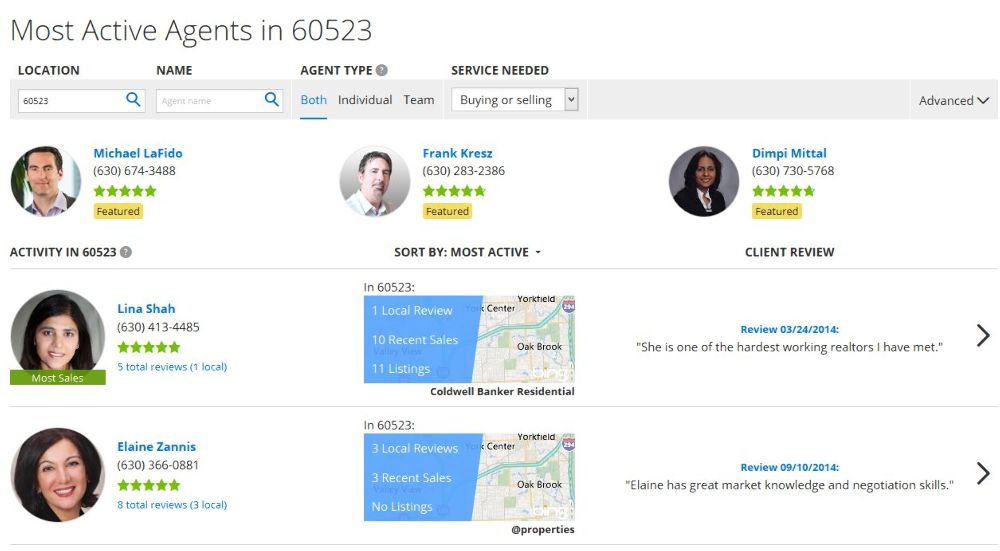In this detailed image, the title "Most Active Agents in 60,523" is displayed prominently in black lettering at the top. Below it, a bold black heading spans from left to right, listing the categories: "Location," "Name," "Agent Type," and "Service Needed."

Under these headings is a gray rectangular bar that runs horizontally. It contains a search icon followed by the text "60513." Next in the bar is another search icon next to the text "Agent Name." Further along, the words "Both Individual Team" are displayed, with "Both" highlighted in blue and underlined. Continuing, it states "Buying or Selling" followed by an "Advanced" option.

Presented next are photographs of five different agents. The first agent is a man named Michael Lafito, whose phone number is provided alongside his five green-star rating. The second agent, Frank Kratz, also has his phone number listed with a five-star rating.

The third agent, Dempy Middle, is similarly featured with a five-star rating and phone number. Positioned to the left of the second row, the fourth agent is Lena Shaw, a woman with black hair, a five-star rating, and her phone number listed. Finally, Elaine Zanis, another woman with black hair, is displayed with her five-star rating and contact information.

Adjacent to Frank Kratz’s listing is a map, which is likewise present underneath Dempy Middle on the right side. Below Dempy Middle’s section, a review reads, "She is one of the hardest working realtors I've met." Beneath Elaine Zanis's entry, another review states, "Elaine has great market knowledge and negotiation skills."